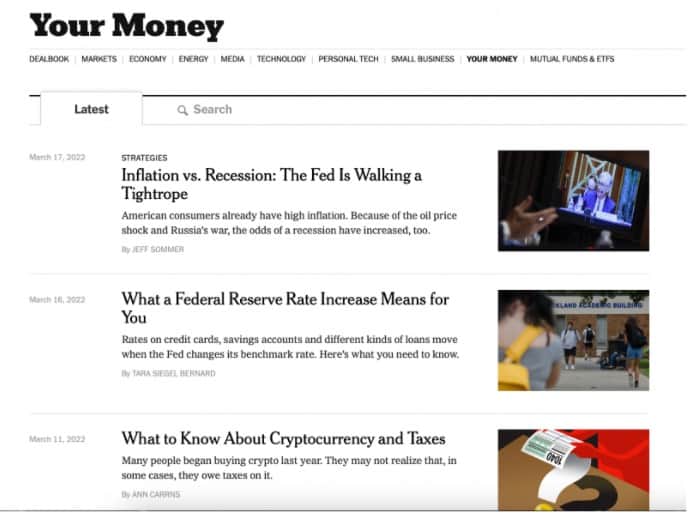Screenshot of a webpage displaying a series of financial articles under the heading "Your Money." At the top left, a navigation menu features multiple tabs: DealBook, Markets, Economy, Energy, Media, Technology, Personal Tech, Small Business, Your Money, Mutual Funds, and ETFs. Below the date "March 17, 2022," three articles are listed under the "Latest" section with accompanying images that correspond to their topics. The first article, titled "Inflation vs. Recession: The Fed is Walking a Tightrope," discusses the delicate balance the Federal Reserve must maintain. The second article, "What a Federal Reserve Rate Increase Means for You," explains the potential personal impact of rate hikes. The third article, "What to Know About Cryptocurrency and Taxes," provides insights into the tax implications of cryptocurrency investments.